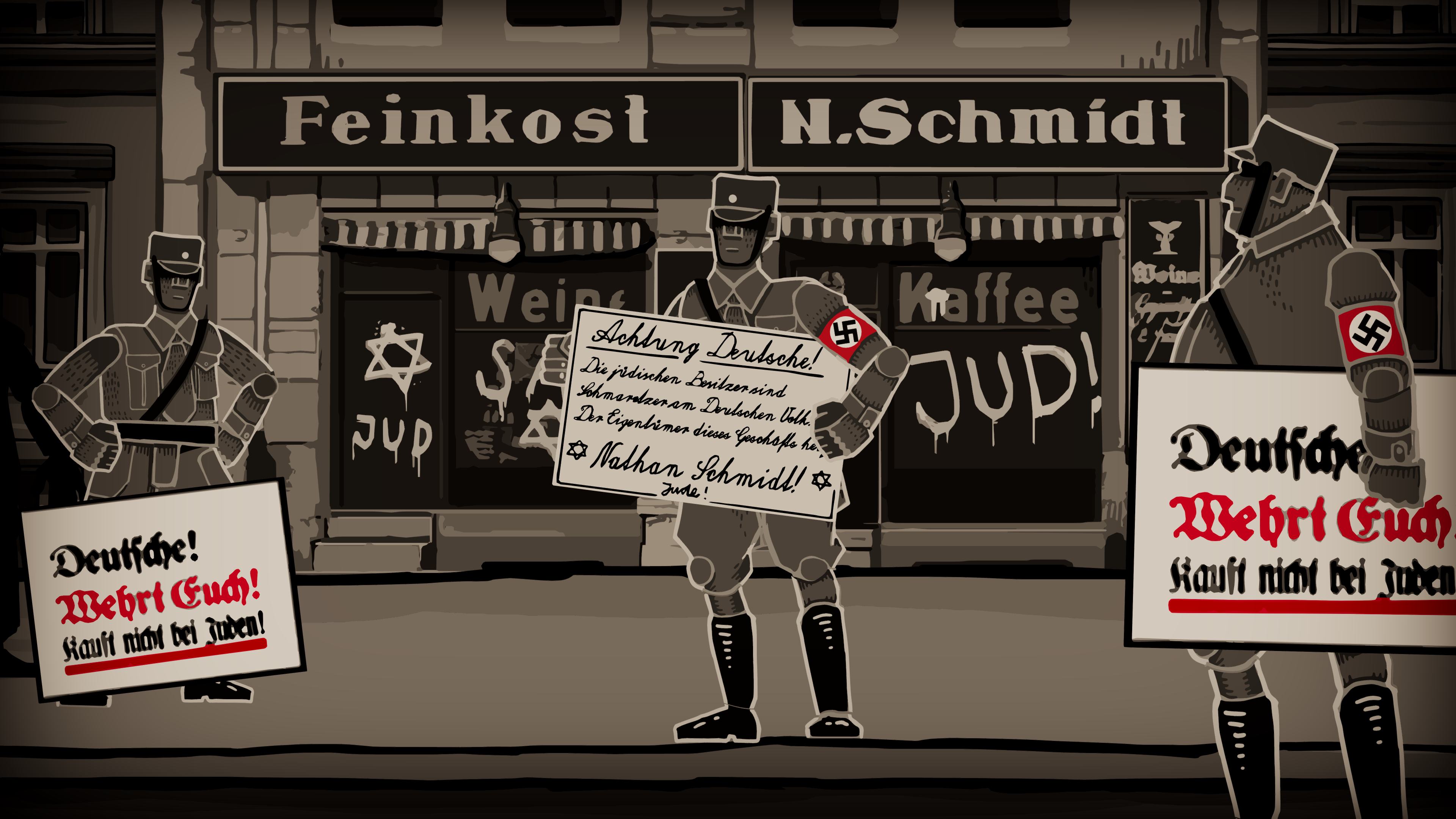The image is a detailed drawing, resembling a cartoon with a construction paper animation style, featuring three Nazi soldiers depicted with human-like proportions. The medium is predominantly black and white with striking hints of red, especially on the Nazi armbands worn by two of the soldiers. They stand in front of a storefront with signage reading "F.E.I.N.K.O.S.T." and "N.S.C.H.M.I.D.T.," which suggests a location in Nazi Germany. The graphic shows the soldiers clad in full military uniforms, including boots and chin-strapped hats. Each holds a sign with German text, but the content of these signs remains unreadable. One soldier has his hands on his hips, gripping a sign, while another holds his sign with both hands, and the third looks to the side while carrying his sign. Behind them, a spray-painted symbol of Judaism is visible on a shop window, hinting at the harassment and anti-Semitic activities they are likely engaging in.